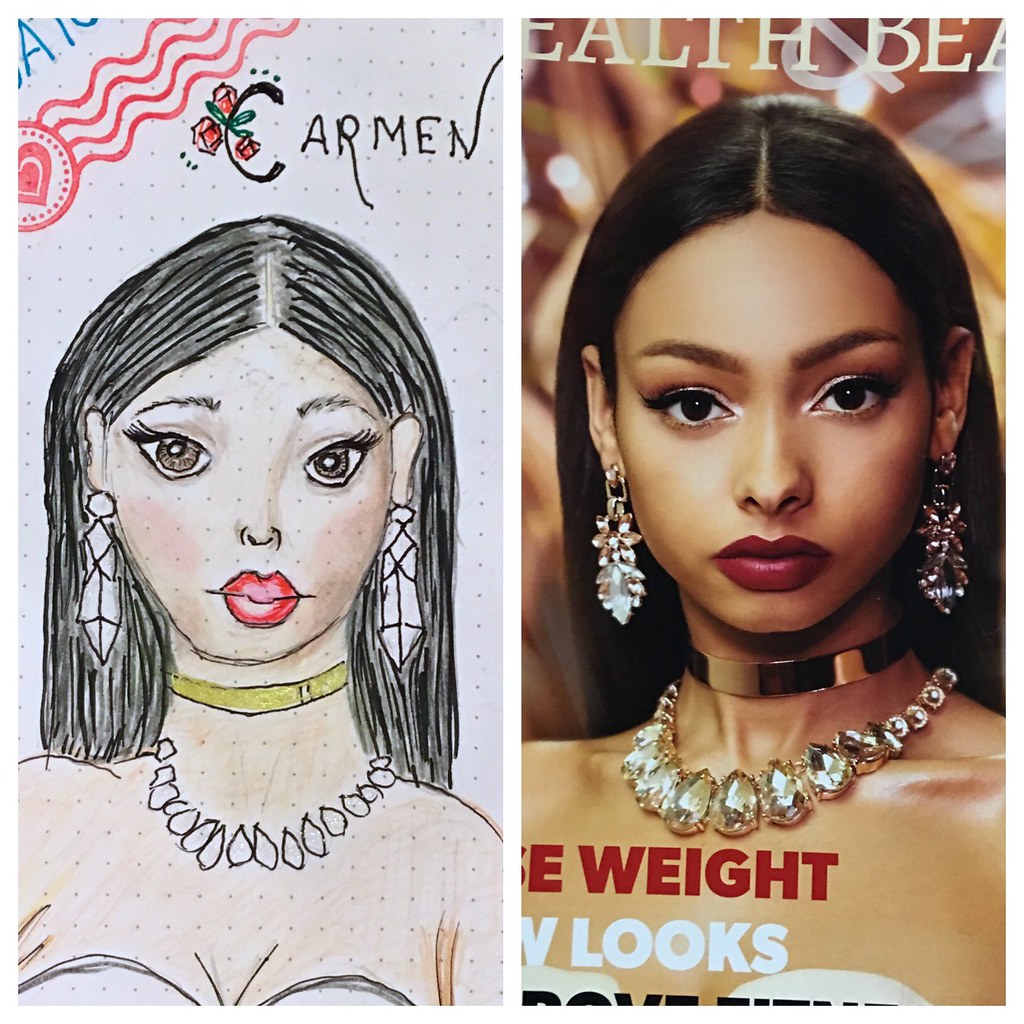The image is a side-by-side comparison of a magazine cover and its drawing. On the right, the magazine cover features a beautiful young woman with long, straight, dark hair parted in the middle, and striking red lips. She has dark brown eyes, accentuated by dusty eye shadow, and dark eyebrows. She dons elaborate rhinestone earrings and a necklace with large teardrop-shaped crystals, complemented by a solid gold choker. Her shoulders are bare, revealing a white, sleeveless garment. The background is golden with a hint of light, and partial text on the cover includes words like "weight" and "looks." The woman appears to be of Latino heritage.

On the left is a hand-drawn illustration of the same woman, titled "Carmen" at the top, with roses encircling the "C." The drawing, executed with paint or markers on a grey dotted background, replicates her long black hair, red lips, and ornate jewelry—including the rhinestone earrings, gold choker, and diamond-like necklace. The artist used yellow to depict the gold choker and pale flesh tones for her skin, adding subtle dots for texture and detail. The name "Carmen" is written in bold black letters above the figure’s head in a whimsical, childlike style.